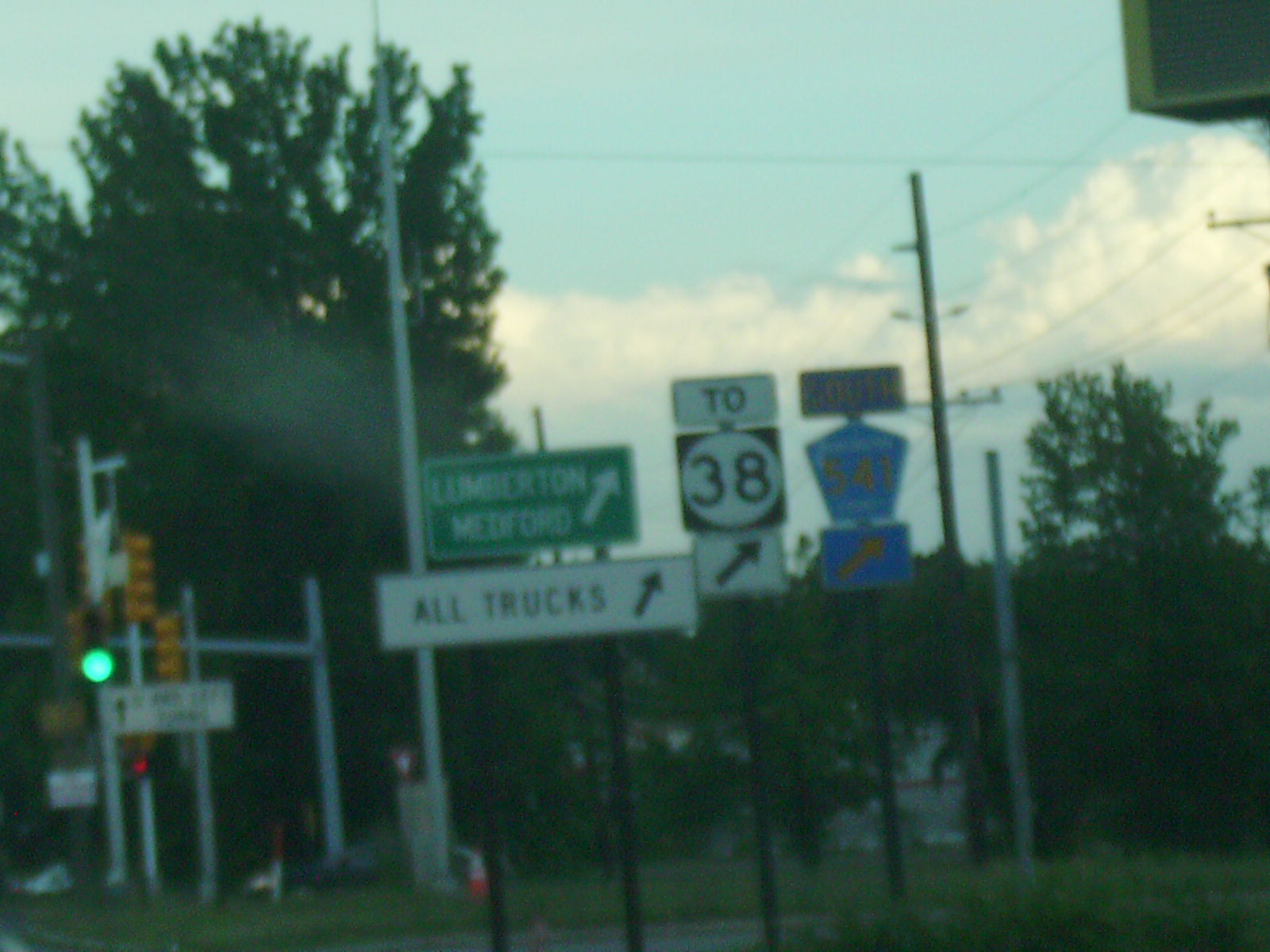A slightly grainy photograph capturing a bustling intersection. At the center, various road signs draw the eye, including a prominent green and white sign and a white and black sign directing "All Trucks" with an arrow. Additionally, a sign for Route 38 with an arrow is clearly visible, alongside a blue sign with brown lettering. Power lines crisscross the scene above a collection of vivid green leafy trees. Patches of blue sky and fluffy white clouds add a serene backdrop to the otherwise busy tableau. On the left side of the image, a traffic light glows green, with a black and white sign positioned below it. In the distance, a red and white road sign is faintly discernible. There is also a distant car near what appears to be a traffic cone, hinting at ongoing road work or traffic control in the area. The image captures a slice of daily life at a bustling crossroad, framed by nature and human activity.